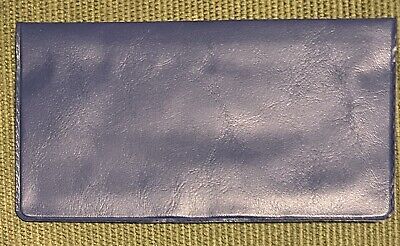The image is of a patent leather checkbook case or billfold wallet, rectangular in shape, measuring approximately eight inches in length and four inches in width. The case is predominantly blue, appearing pale blue under the harsh, bright light that creates strong highlights and shadows across its shiny surface. The lighting could be from a camera flash or intense overhead light. The texture of the background fabric, which supports the case, is noticeable; it is a gold or brownish-green woven material with shimmery strands, reminiscent of burlap or straw, adding a patterned texture to the scene. The checkbook case appears empty, with no contents visible inside.